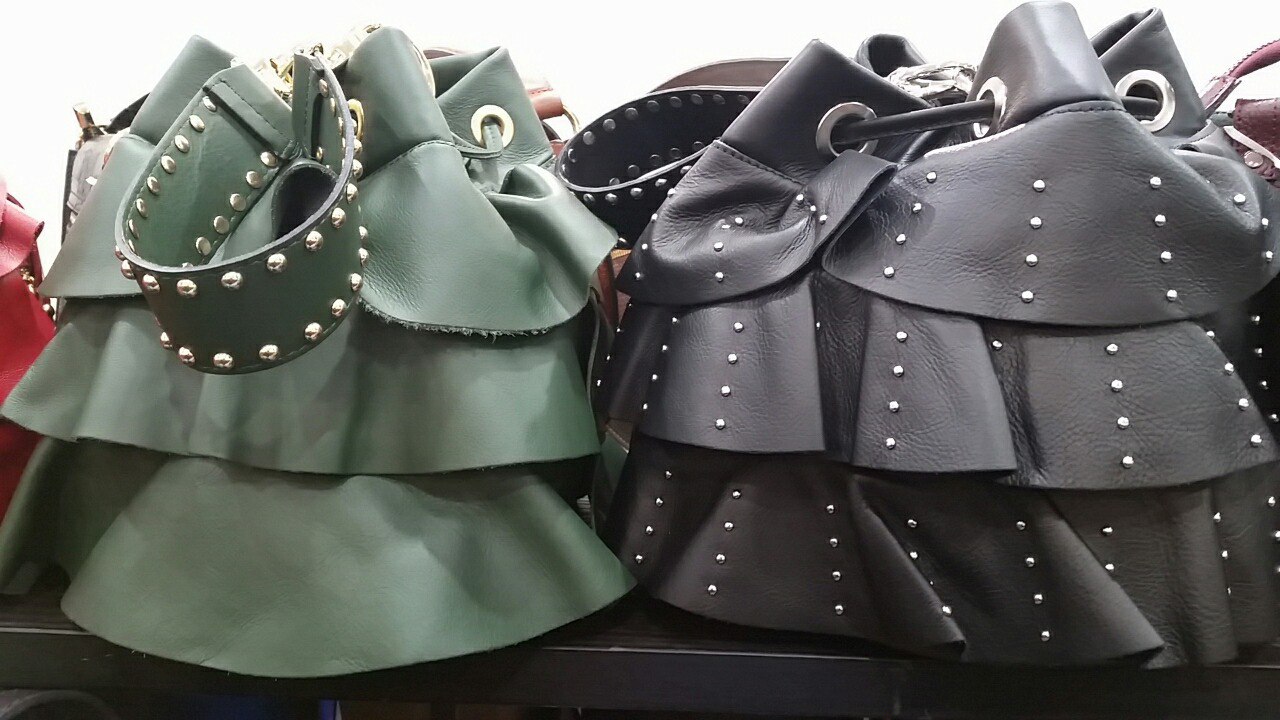This high-resolution, color photograph showcases a detailed close-up of two centrally-placed handbags, positioned against a stark white background under bright lighting. Both handbags share a similar layered design, reminiscent of a ruffled skirt, each with three distinct layers. The bag on the right is black, embellished with studs that mimic white diamonds along each ruffle, and features large silver loops at the top, suggesting it might be a drawstring closure like a backpack. Its strap resembles a studded belt, adding to the intricate detailing. The bag on the left is a muted military green, also layered but without the gemmed studs, maintaining an elegant simplicity with similar flaps and silver rings at the top. Additional handbags in shades of red, maroon, and brown can be partially seen in the background, hinting at a diverse collection possibly displayed for commercial purposes, like on a retail site.